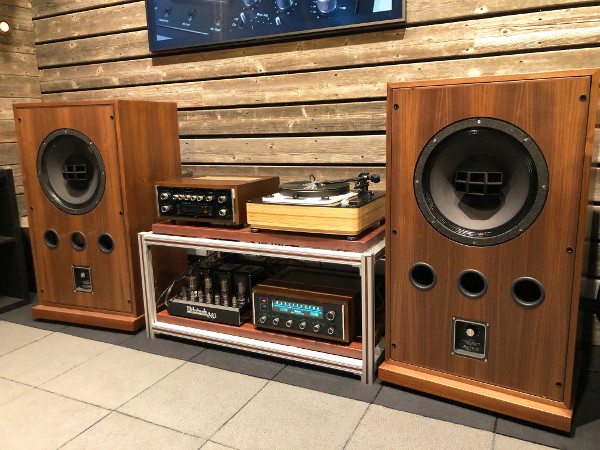The image depicts a home audio setup set against a visually appealing shiplap wall made of wooden slabs. Central to the arrangement are two large, wooden stereo speakers with black sound outputs, positioned on either side of a compact entertainment center. This center structure, which sits directly on the tiled floor, features a series of audio equipment that includes a light wood-grain turntable with a record on it, situated at the top. Directly beneath the turntable are two receivers, both equipped with various knobs and switches for controlling audio playback. The bottom left receiver is notable for its blue-lit display showing radio frequencies. Additionally, on the bottom shelf next to the receivers, there is a black device with more controls. Above the entire setup, a flat-screen TV is mounted on the shiplap wall, completing the entertainment ensemble.